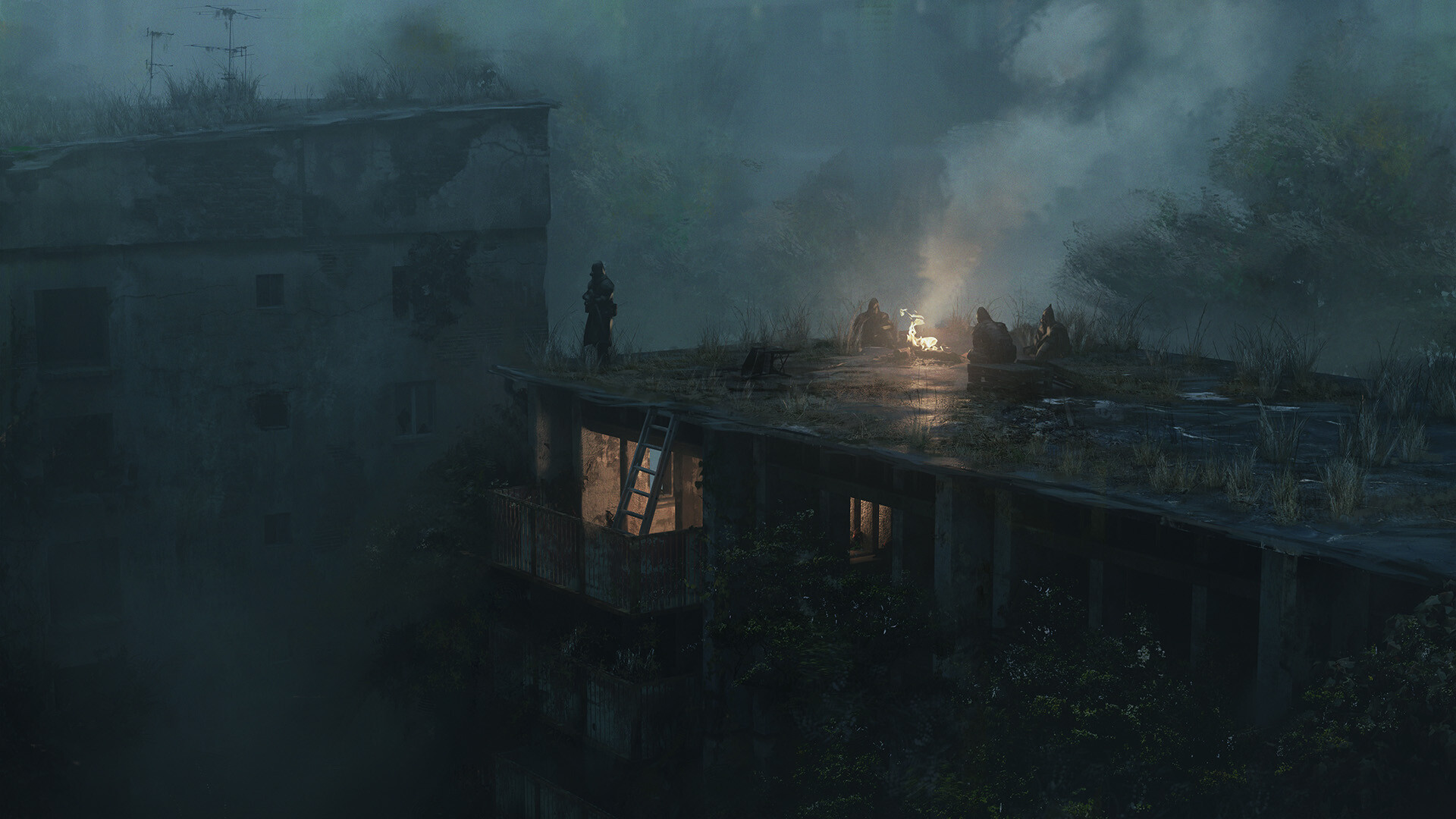The image depicts a stylized piece of concept art, likely intended for a movie or video game reminiscent of "Elden Ring" or the "Dark Souls" series. The scene captures an eerie, nocturnal atmosphere with heavy fog and limited visibility. Four figures, presumably soldiers or explorers, gather atop a decrepit, overgrown building. Three of them sit close together around a fire, the flickering flames sending tendrils of smoke skyward, while the fourth figure stands apart, perched on the edge of the building, gazing out into the obscured distance.

The environment exudes abandonment and decay; vines and dying plants crawl over the structure's surfaces, hinting at long-forgotten times. A rickety ladder descends from the roof into a dimly illuminated room within the building, suggesting hidden spaces and potential secrets below. In the hazy background, another dilapidated structure looms, shrouded in the same thick fog that blankets the scene.

This setting evokes a sense of suspense and stealth, as though it's a moment of respite for these figures amidst a perilous journey. The overall dark, foggy ambiance and overgrown architecture create a perfect backdrop for a stealth sequence where one might sneak around unseen foes, adding layers of tension and intrigue to the visual narrative.